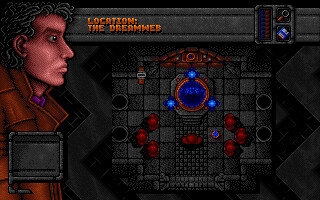The image showcases a dynamic scene centered around a black and gray checkerboard or chessboard, scattered with vivid red figures positioned at various places on the squares. To the side of the board, a man is visible from the torso up, standing in profile. He has white skin and curly grayish hair, and wears a classic brown trench coat. His face is oriented straight ahead, his expression contemplative. A gray banner overlays his face, inscribed with the text "Location: The Dream Web" in bold orange letters. The background features a distinctive zigzag pattern in shades of gray and black, adding a surreal, dream-like quality to the composition.